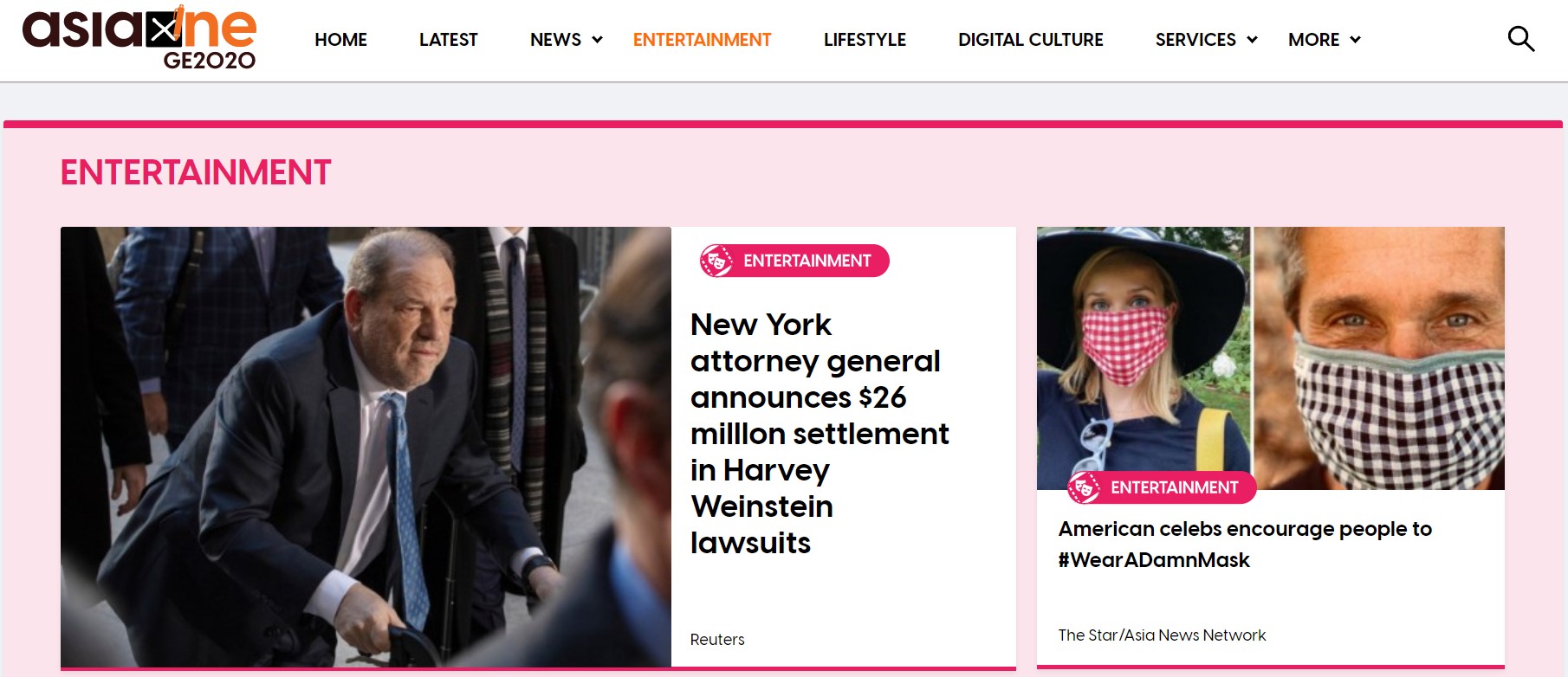The screenshot depicts a web page against a plain white background. At the top, a white header features "Asia" in bold black text, with the letters "I" and "E" in red, followed by "GE 2020" in smaller black text below. The navigation menu spans the header in black text and includes options such as "Home," "Latest," "News" with a pull-down arrow, "Entertainment" (highlighted in red), "Lifestyle," "Digital Culture," "Services" (with a pull-down arrow), and "More" (also with a pull-down arrow).

The page focuses on the "Entertainment" section which is marked by a red label on a pink background. The prominent headline announces, "New York Attorney General announces $26 million settlement in Harvey Weinstein lawsuits." To the left of the headline, there is a color photo of Harvey Weinstein. He is depicted wearing a blue suit and tie, using a walker for support.